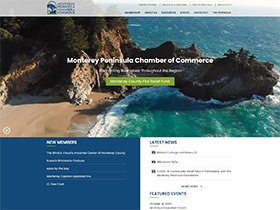This tiny screenshot captures a vivid aerial view, presumably taken by a drone, showcasing a picturesque lagoon by a beach. The central image displays a striking rock formation extending into the greenish-blue water, with beige sand and frothy white waves washing up on the shore. The scene is bathed in sunlight, casting shadows from the rocks, highlighting the natural beauty of the area on what appears to be a bright, sunny day.

Above the image, there is a semi-transparent, off-white overlay with text, which remains largely unreadable due to the small size of the screenshot. However, the main visible text within the picture reads "Monetary Peninsula Chamber of Commerce," followed by smaller, white text, and a green rectangular button with white text, though the specifics are indiscernible.

Beneath the main image are two text boxes: a blue box on the left and a white box on the right, both containing text that is also unclear in this minute screenshot.